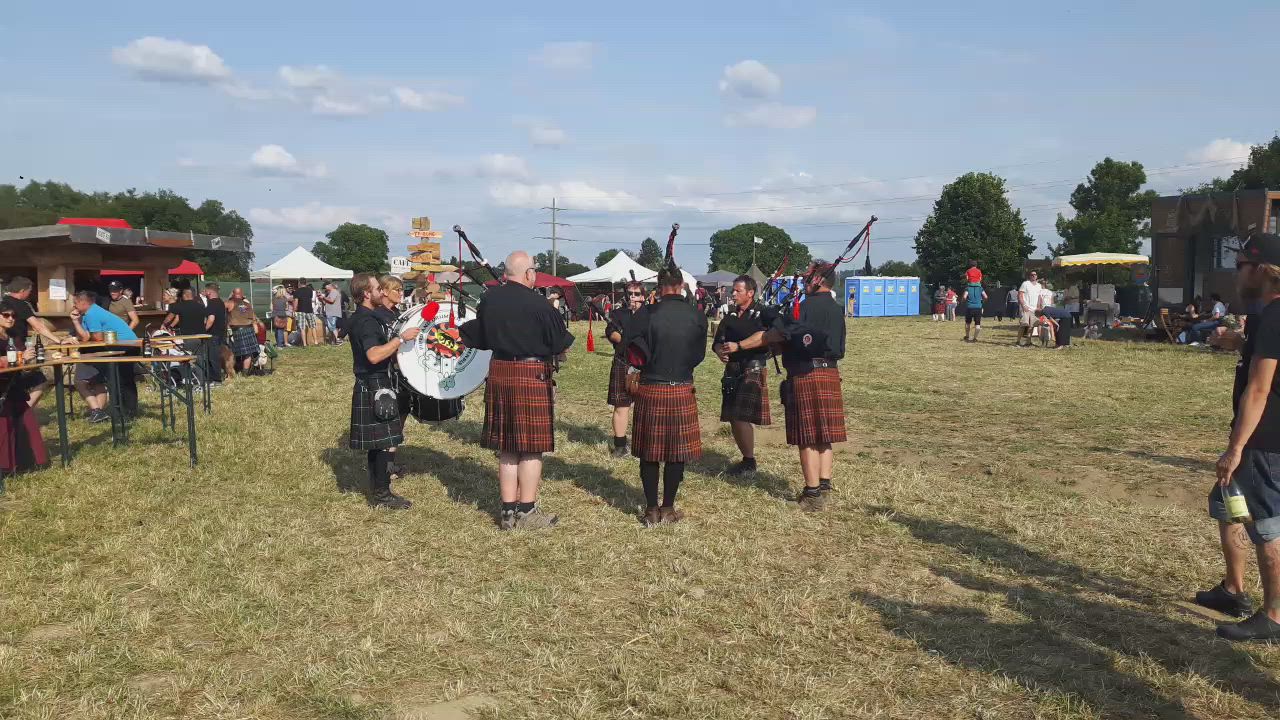Captured amidst a field of patchy, greenish-brown grass, this vivid outdoor photograph showcases a lively festival scene. In the center, a group of men clad in traditional kilts are performing music; most sport red checkered knee-length kilts, with one in green, all complemented by black button-up shirts. They stand in a circle, engrossed in their performance with bagpipes and a side drum. Surrounding them, people are seated on chairs and at outdoor tables, likely enjoying the music or conversing. The backdrop reveals various open-air tents with cloth roofs, scattered trees near the horizon, and a line of blue port-a-potties to the far right. The sky above is a clear blue adorned with a few clouds, perfectly framing this vibrant outdoor gathering.